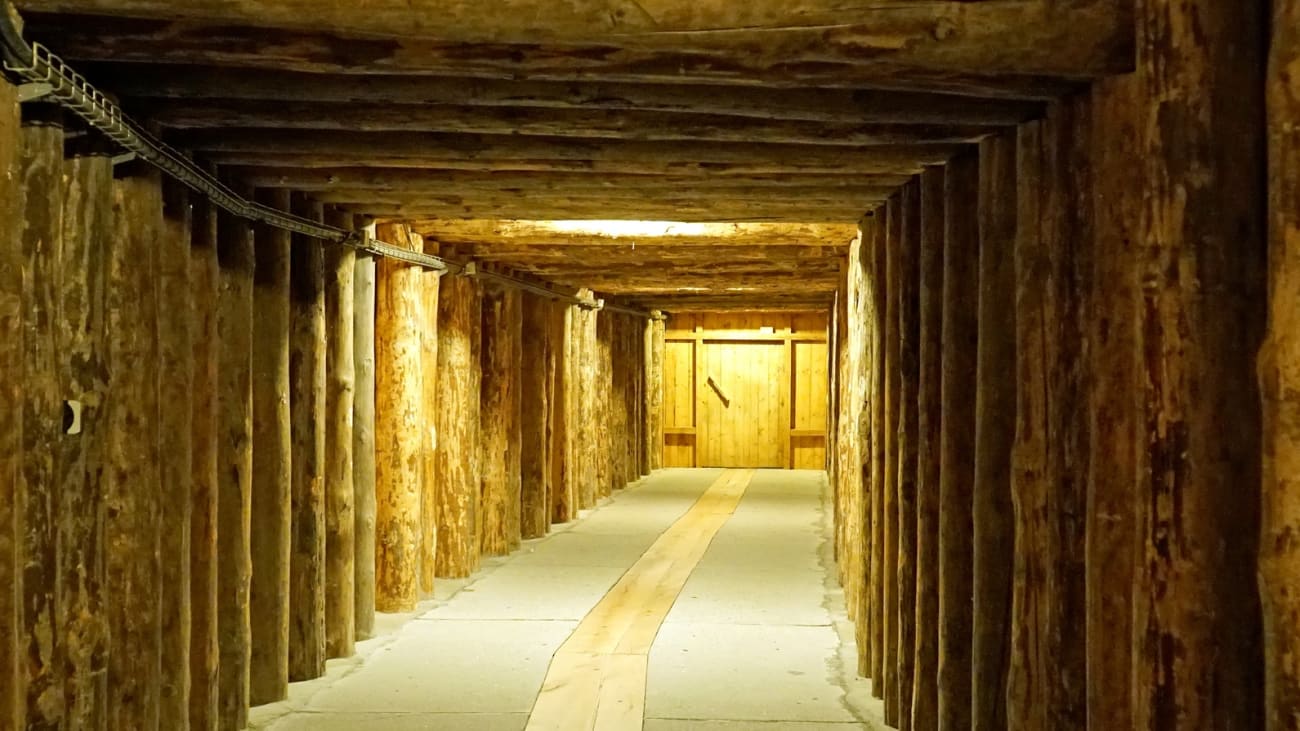This image depicts a long, narrow passageway that appears to be part of an underground bunker or a house under construction. The tunnel is lined with wooden planks on both sides, creating a rudimentary, somewhat eerie atmosphere. The wood exhibits rich tones of brown, orange, and yellow, adding to the rustic feel. On the right side, metal brackets run along the length of the tunnel, possibly supporting the wooden walls. The ceiling has a grid-like structure made of wood, and there is a hint of insulation visible near the top. 

A partially concrete floor, in a yellow-gray hue, forms a path that guides the eye to a large wooden door at the end of the passage. The door is framed by additional wooden slats and has a handle on the left side. Ambient yellow light illuminates the scene, with some natural sunlight peeking through a break in the wood above, contributing to the otherwise dim lighting. This setup, devoid of any signs or markings, gives off a bit of a creepy, abandoned vibe.